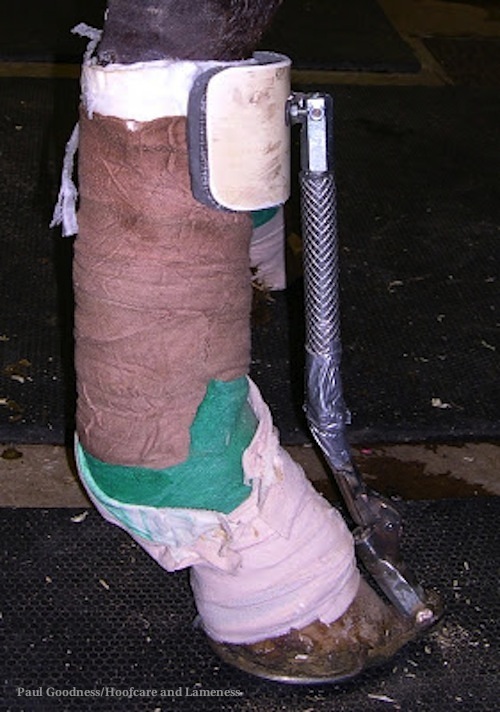This image appears to depict the side view of a horse's leg encased in a multi-colored cast and supported by a mechanical brace. The leg is bandaged in a wrap of white, green, and brown colors. The metallic reinforcement rod of the brace extends from the hoof up to about one foot along the leg, featuring a semicircular attachment at the top. This rod serves as a structural support, connecting to a partial wraparound plastic piece that ensures stability. The entire setup is placed on a dark, possibly rubber-matted, surface. On the bottom left of the image, there's a small, legible inscription that reads "Pull Goodness / Hoof Care and Lameness." This seems to suggest that the image is related to veterinary care for horses with leg injuries. The overall background of the image is very dark, making the leg and its supportive apparatus the focal point.